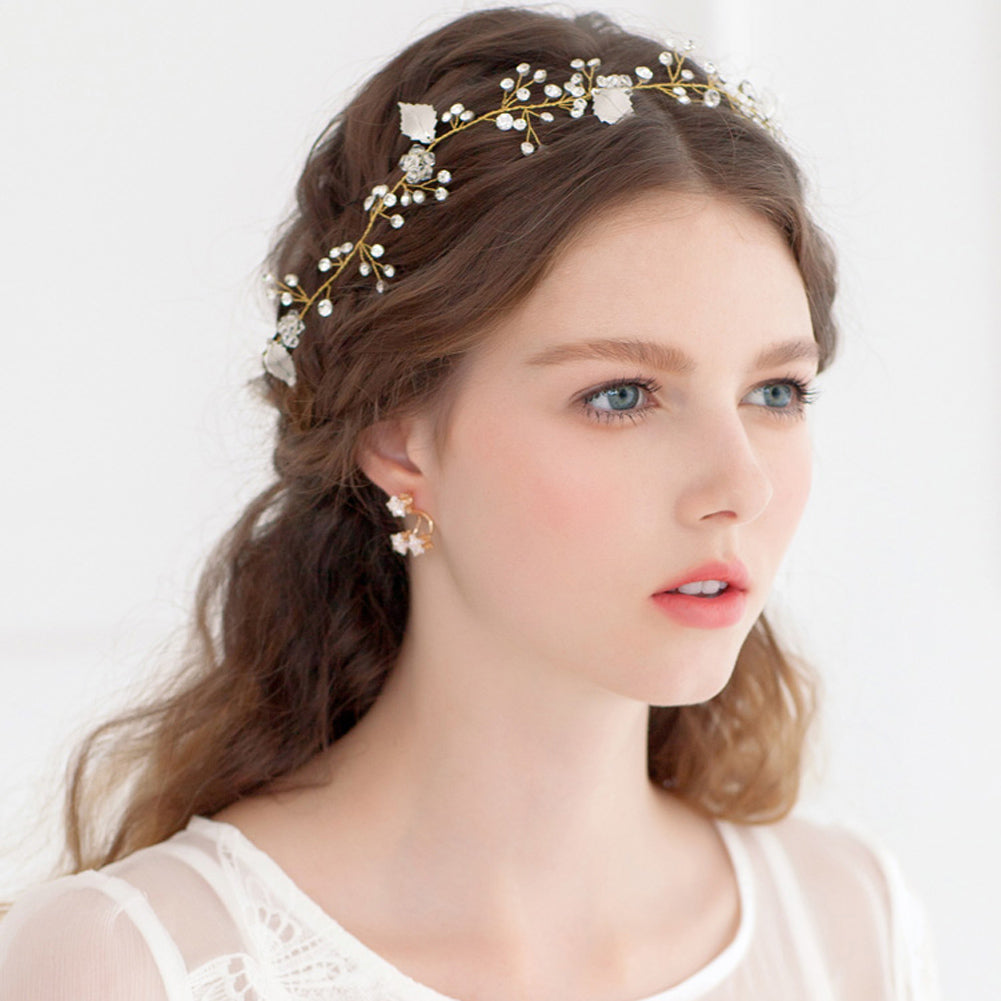This image captures a striking, possibly AI-generated or highly professional portrait of a young, white female model or bride. The background is a plain, white studio setting, ensuring all focus is on the subject of the image. She has captivating blue or aqua green eyes, and her gaze is directed sideways towards something out of frame. Her lips are painted a delicate pink, complementing her shoulder-length, brown hair which is elegantly adorned with a beautiful hairband or crown. This headpiece features an intricate design of flowers, leaves, and small buds, likely crafted from diamonds or pearls. Adding to her regal appearance, she is wearing earrings shaped like three stars. The photograph highlights her flawless makeup, enhancing her already striking features, and she is dressed in a white gown, although the image is cropped at the neck, focusing solely on her facial features and accessories.